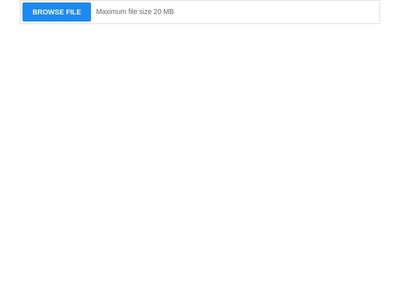The image features a user interface element with a white rectangular box bordered in gray on all four sides. Positioned on the left within this box is a dark blue rectangle. Inside the blue rectangle, centered in bold white capital letters, is the text "BROWSE FILE." To the right of this blue rectangle, in small light gray letters, is the note "Maximum file size 20 MB." The overall design is minimalist, providing clear instructions and limitations for file browsing and uploading.